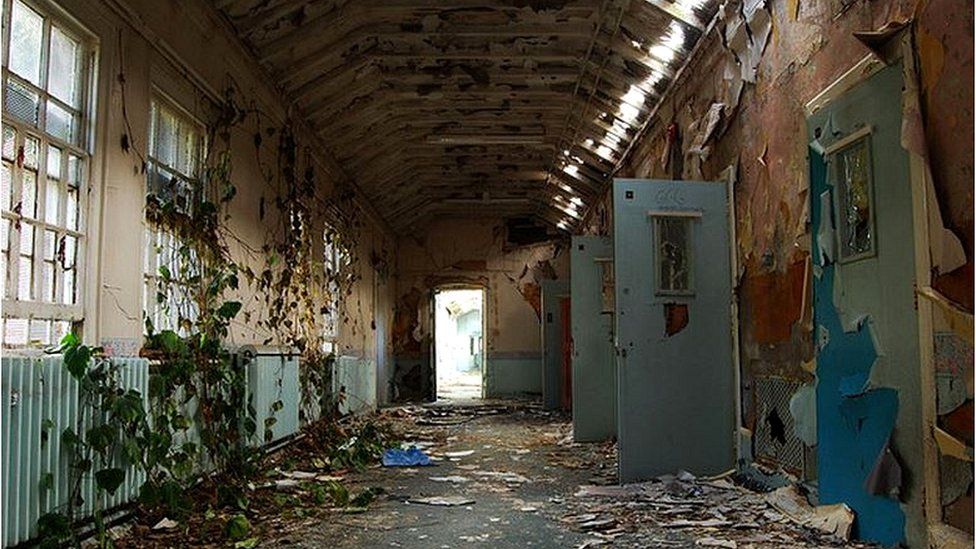The image depicts a long, dilapidated hallway of an abandoned building, possibly a prison, hospital, or schoolhouse. The floor is cluttered with dirt, broken roofing, and wall debris, contributing to the overall desolate atmosphere. On the left-hand side, large, multi-paned windows painted white but now peeling, allow ample light to stream in; some have mesh screens or bars, indicating a previously secure environment. Ivy with large leaves grows from the floor to the ceiling, even crawling over the old radiators lined along the wall.

On the right-hand side, a series of metal doors—three visible open and one closed—are spaced evenly along the peeling gray-to-blue walls. These doors are equipped with narrow, square windows, some with broken glass, suggesting a utilitarian design. An air return vent is positioned between the front two doors. Overhead, fluorescent light fixtures hang from a cracked and peeling ceiling that narrows toward the top, creating an almost claustrophobic feel. At the end of this haunting corridor, an open door reveals a flood of sunlight, offering a stark contrast to the dark, deteriorating interior.